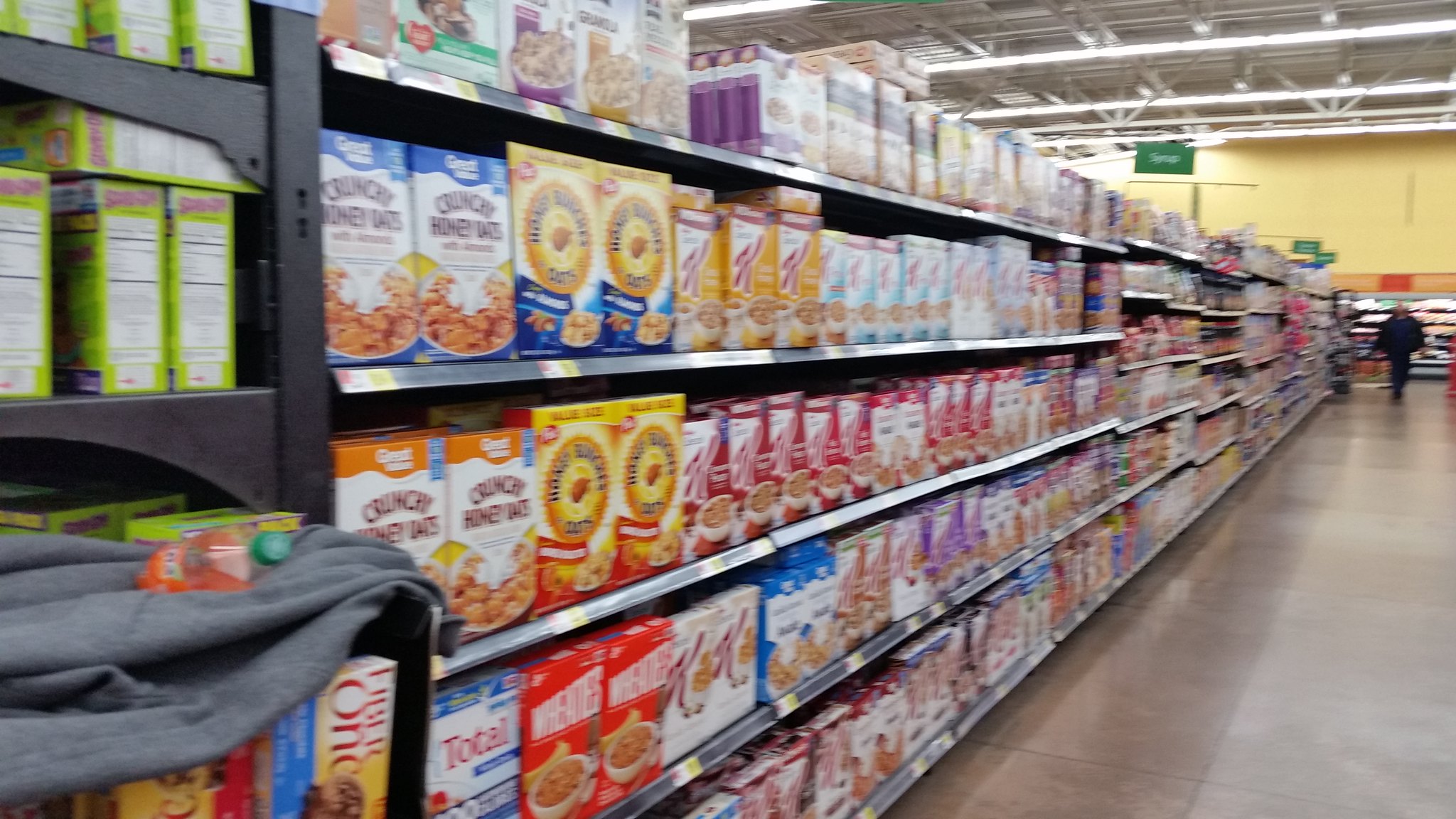In the image, we observe the interior of a store. The foreground features an aisle laden with various items, organized on shelves. In the background, a person is captured mid-stride, contributing to the bustling atmosphere. The ceiling, visible in the top right corner, is adorned with a network of silver pipes and wires, giving the store an industrial feel. The back wall is painted a vibrant yellow, adding a splash of color to the scene. On the top left side of the image, there is a conspicuous black shelf holding light green boxes, further emphasizing the store's orderly arrangement of goods.